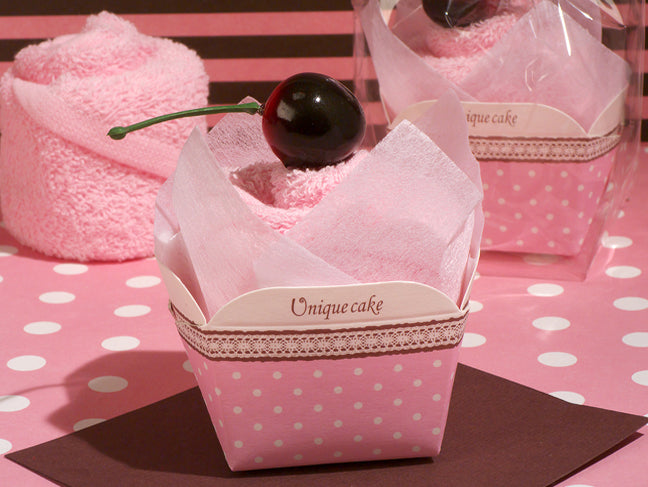The image captures a landscape-oriented photograph featuring a whimsical pink-themed setup. At the center is a paper container reminiscent of a Chinese takeout box, adorned with pink and white polka dots, a red and white lace trim, and inscribed with the phrase "unique cake" in brown. Inside the container, there appears to be a folded pink towel cleverly styled to resemble a pastry, crowned with a deep red cherry. The package rests on a deep red/brown cocktail napkin, which sits atop a pink tablecloth dotted with white spots. In the background, another similar container, wrapped in plastic, is positioned to the back right and a folded pink towel is visible in the upper left. The backdrop features a matching red/brown and pink striped wall, enhancing the cohesive color scheme of the scene.